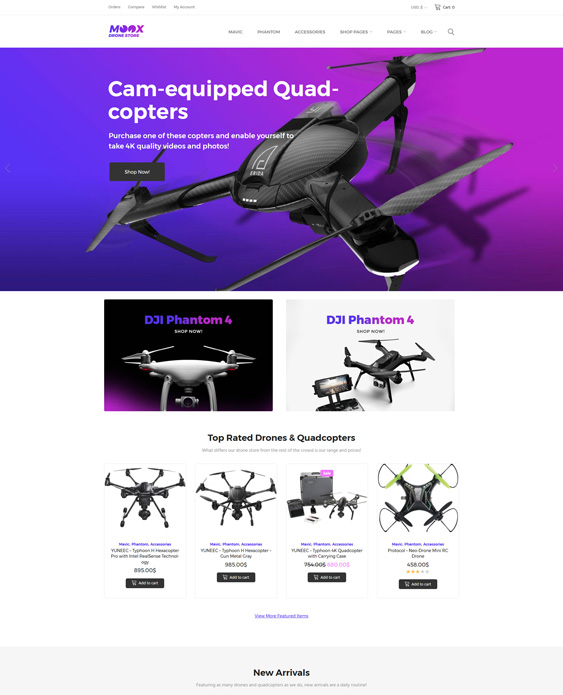The image features a white border at the top and is significantly blurry and small, making most text illegible. Below the white border is a purple section displaying an image of a drone with the caption "Cam equip quadcopters." The drone is black with three wings and propellers. Beneath this image is a box displaying another drone labeled "DJI Phantom 4." A similar box to the right showcases a different colored version of the DJI Phantom 4. Underneath these, there is a section titled "Top Rated Drones and Quadcopters" showcasing four different drones. Each drone is accompanied by blue text and black text, and there is a black button below each drone. At the bottom of the page, there is a blue hyperlink labeled "New Arrivals," followed by extensive white empty space.